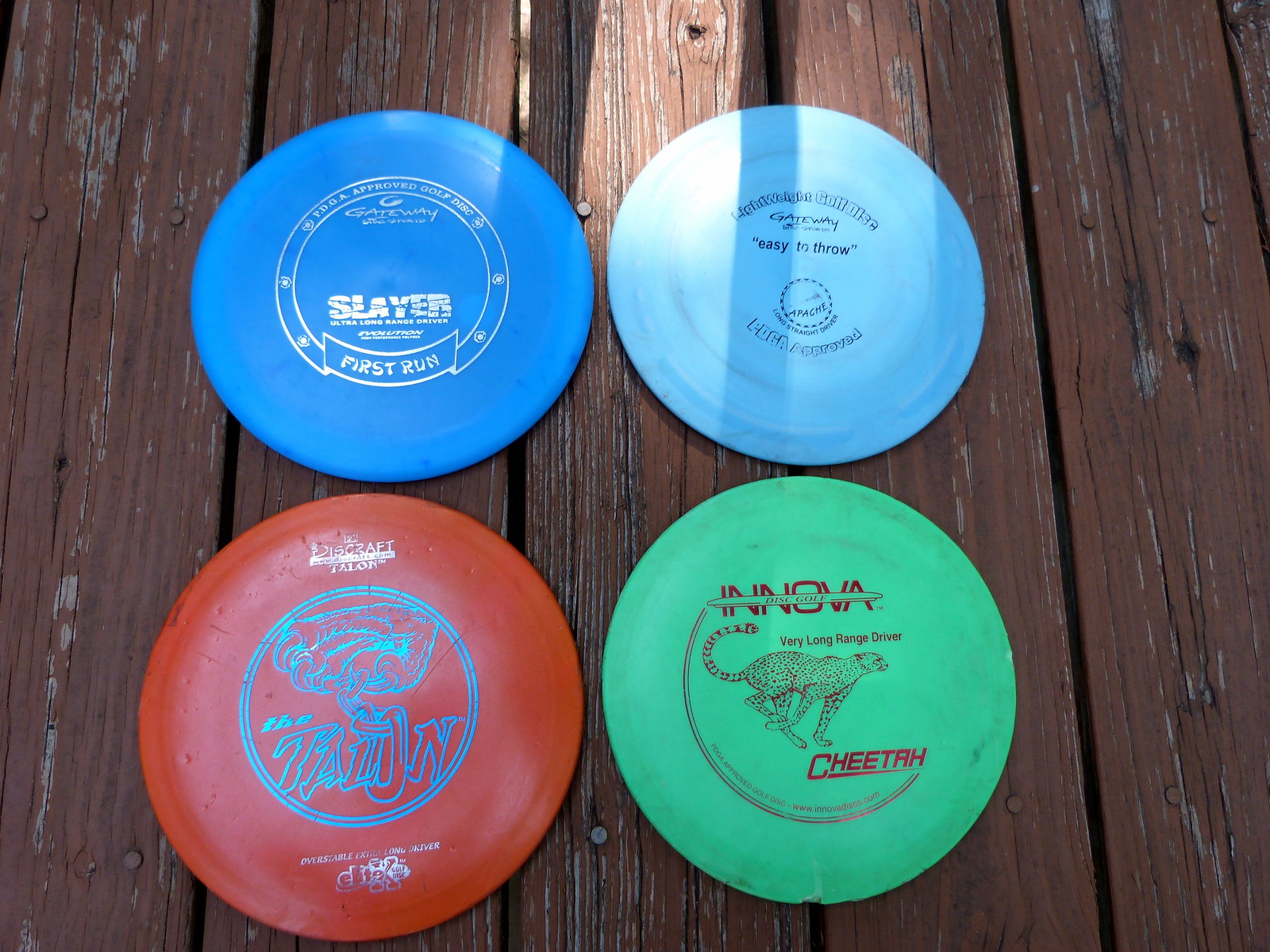The image displays four colorful frisbees methodically arranged in a square formation on a weathered wooden deck with brownish-red slats that are starting to peel. The top row features two blue frisbees: the upper left one is a dark royal blue marked with "FPGA-approved golf disc, Gateway Slayer, first run" along with some unreadable smaller text, while the upper right one is a lighter baby blue inscribed with "Lightweight Golf Disc, Gateway, 'easy to throw,' PDGA-Approved." In the bottom row, the left frisbee is red, labeled "Disc Craft Talon, trademark" with a distinctive double circle in the center containing a drawing of a raptor's foot clutching the 'O' in 'Talon.' Additional text in silver, potentially reading "Elite X," is also present but not clearly legible. The bottom right frisbee is a sea-green color, featuring the brand "Innova, I-N-N-O-V-A, Disc Golf" and the description "Very Long Range Driver" along with an image of a running cheetah and the word "cheetah." All the frisbees exhibit signs of use, with evident scuffs, markings, and dirt, particularly pronounced on the red and green discs.